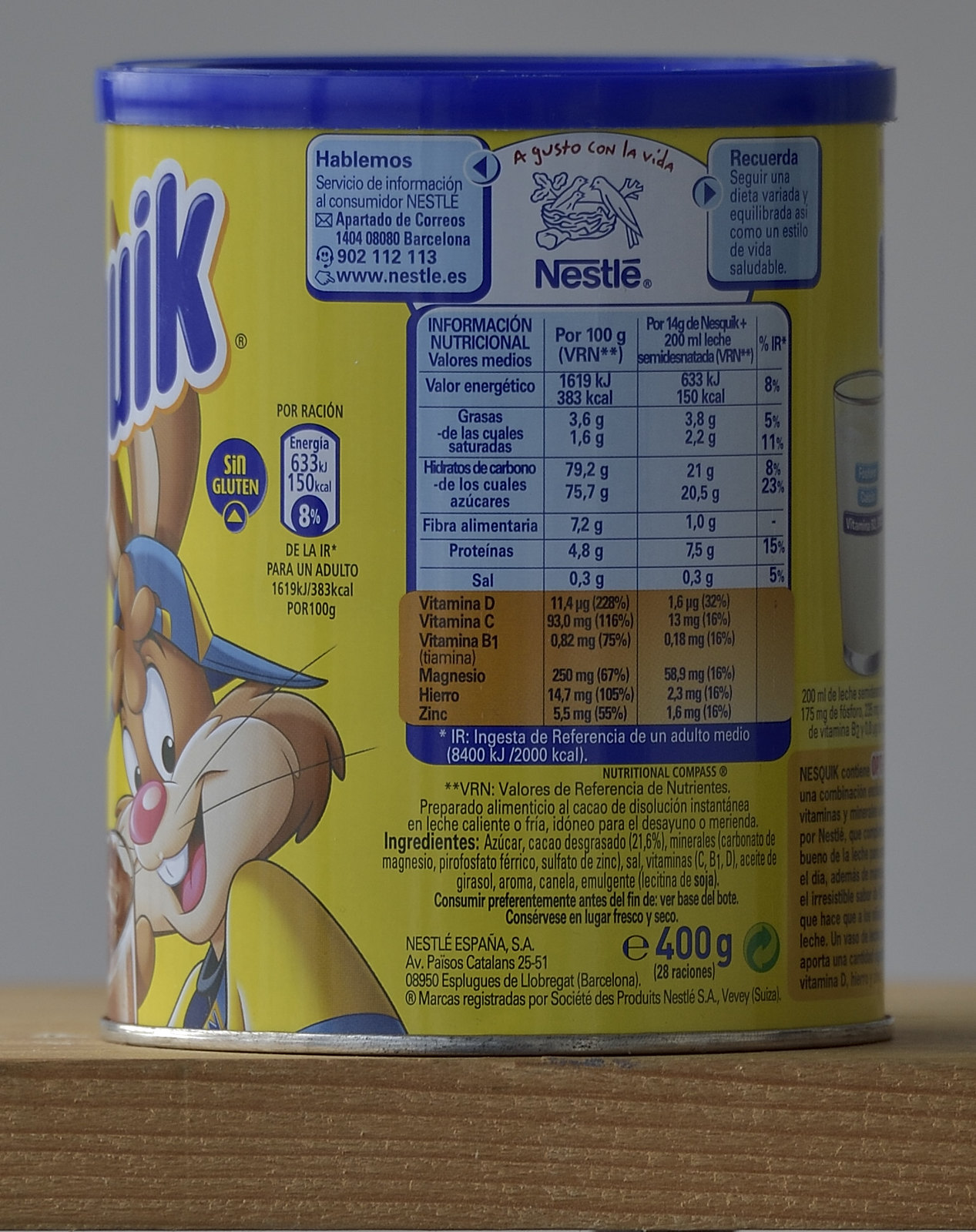This is an image of a can of Nestlé's Nesquik, featuring a bright yellow background and the beloved Nesquik Bunny prominently displayed. The bunny is depicted with large oval eyes, a pink nose, and a pink tongue. He is grinning widely, showcasing his distinctive two front teeth. Dressed in a vibrant yellow and blue outfit and sporting a backwards baseball cap, the bunny exudes an energetic and playful vibe.

The label on the can is in Spanish and displays the Nestlé brand name prominently. Additional blue labels are visible, providing contact information and nutritional facts in clear detail. Despite the text being in Spanish, key nutritional information is listed, including values for fiber, protein, vitamin D, vitamin C, vitamin B1, magnesium, and zinc, all shown in English.

The can also indicates a net weight of 400 grams. On the right side of the label, there is an image of a glass filled approximately halfway with a beverage, suggesting the product's use as a drink mix. The overall design of the can is both informative and visually appealing, catering to both brand recognition and consumer awareness.